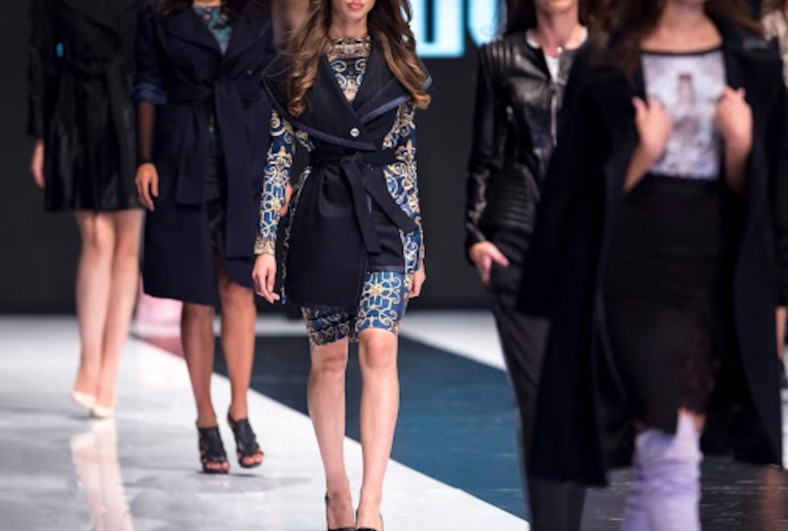In this realistic photo from a fashion show runway, five women, presumably models, are walking in line. The scene is dominated by predominantly black outfits, each distinct in design, highlighting the unique style of each model. The leading model, positioned at the forefront, sports thigh-high purple boots and wears her coat draped over her shoulders like a cape, clutching it at her chest. Behind her, another model in a leather shirt is notable for bold details that suggest androgyny or transgender identity, featuring an accentuated bulge at the waist. The third model displays a form-fitting outfit that mimics tattoos with swirly white symbols on a blue background, leaving her lower legs bare. All models showcase bare skin from the thighs down, adding to the aesthetic appeal. Characters include long, wavy hairstyles and a mixture of high heels in black and white, enhancing the striking contrast against the runway's blue-tiled center flanked by white tiles. The cohesive yet varied fashion choices underscore the creative expressions being paraded down the catwalk.